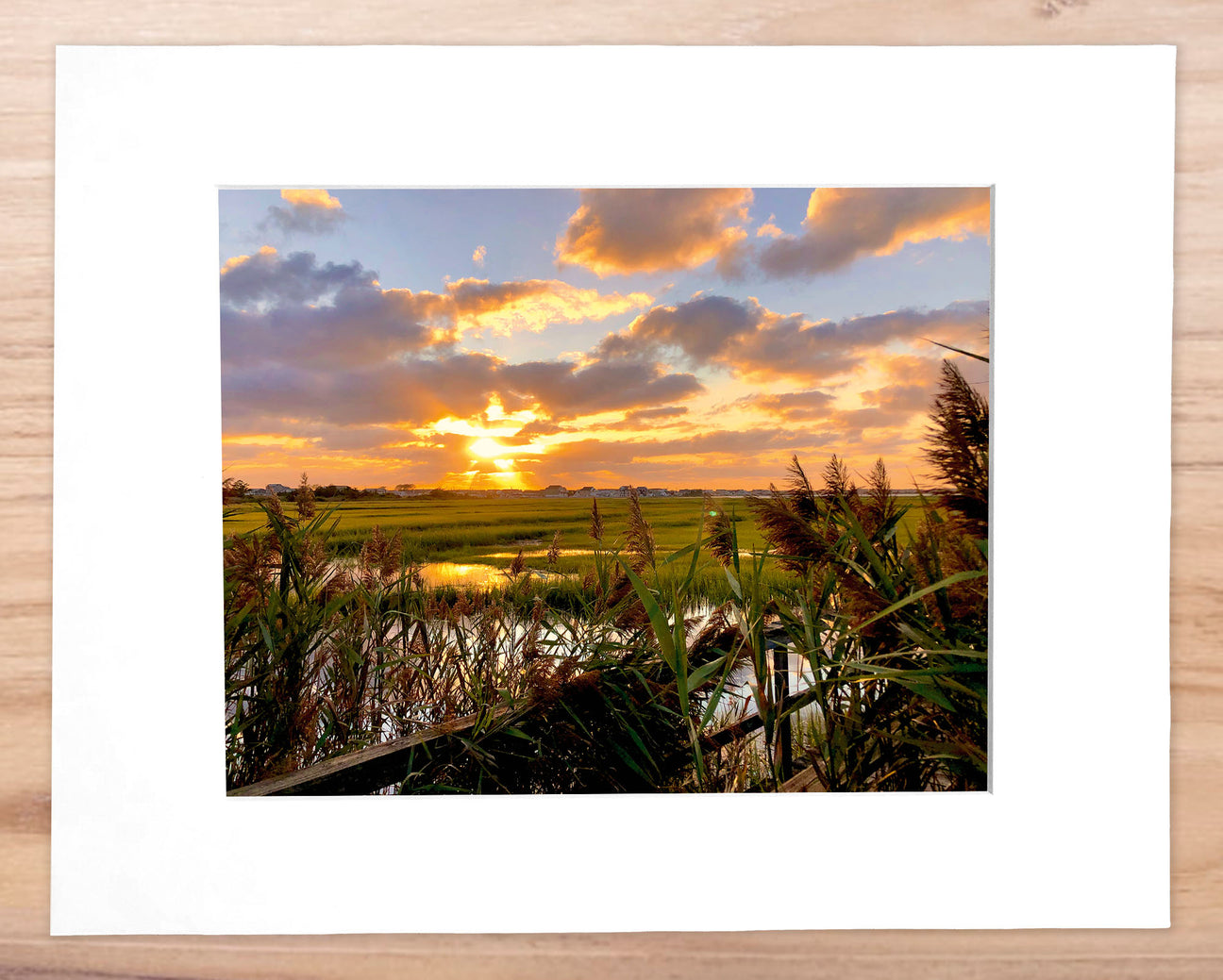This image, likely a stock photo or framed artwork, is set on a wooden oak table. It features a rectangular photo frame approximately six inches wide and five inches high. The frame has a light-colored wood border about a quarter to a half-inch thick, followed by a plain white inner border about an inch wide. The photograph itself, around three inches wide and two to two-and-a-half inches tall, captures an outdoor scene.

The image depicts a marsh or wetland at sunset, viewed from a perspective resembling a walk bridge. The scene showcases a tranquil body of water surrounded by tall grasses, including cattails and possibly pompous grass with wispy flowers at the ends. The sky is split between the top and bottom halves of the photo; the top half features an expanse of blue transitioning to orange and gray as it meets the horizon. Puffy clouds, colored by the setting sun in shades of orange, yellow, and gray, enhance the serene atmosphere. The foreground contains a fenced area that adds a subtle but distinct element to this picturesque and calming landscape. No people or buildings are visible in the photo.